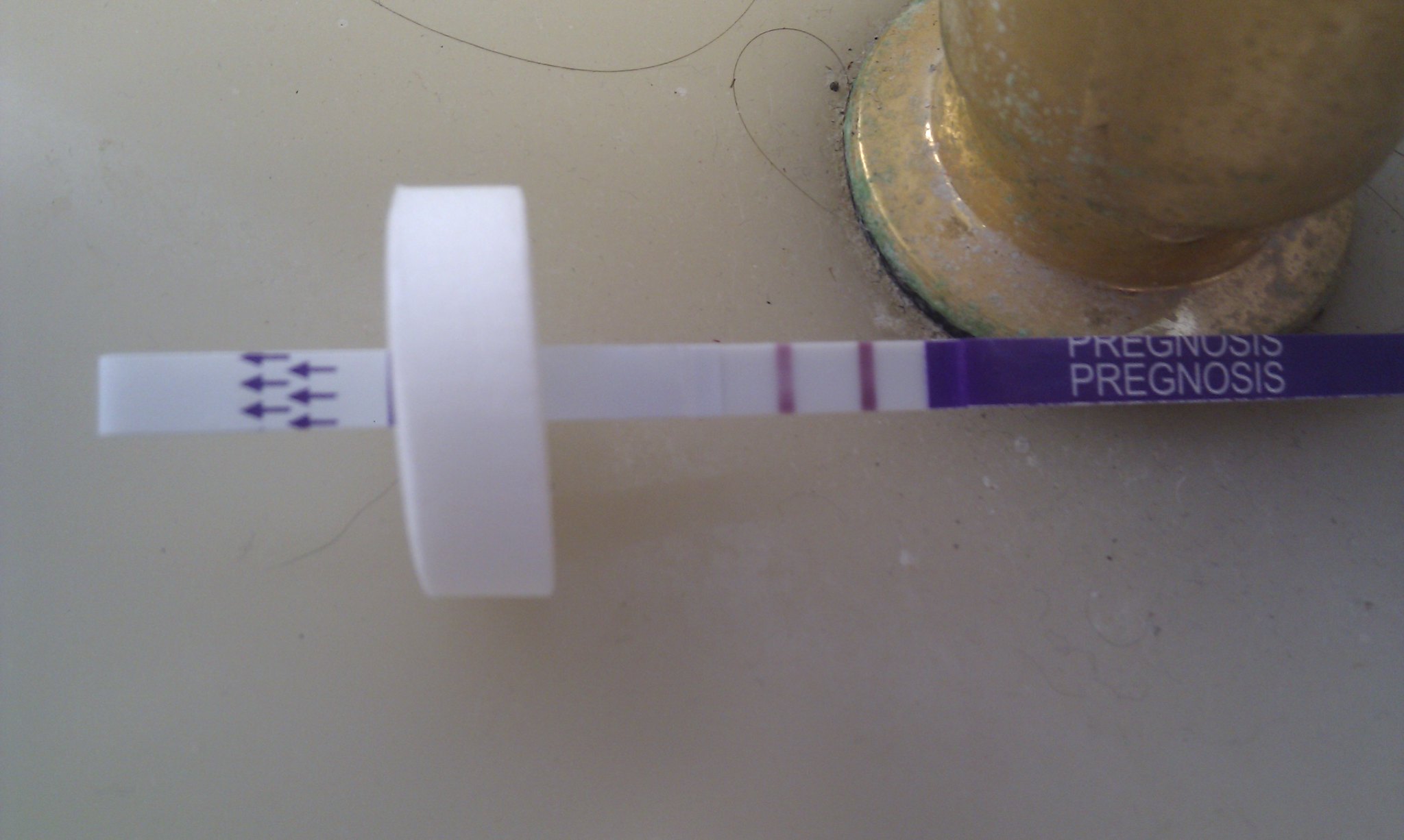The image depicts a weathered, golden-brown doorknob, located in the top right corner, lying flat against a white surface. Only half of the doorknob is visible, revealing significant dust and rust accumulation. Surrounding the doorknob, green algae or mold scatters alongside various hairs, some of which form a U-shape near the top of the image. Below the doorknob, a white tube with a purple label prominently features the word "prognosis" circling around it. The tube also has two pink lines next to the purple label. On the left side, there are purple arrows pointing left, and a white cap encloses the tube at the bottom.